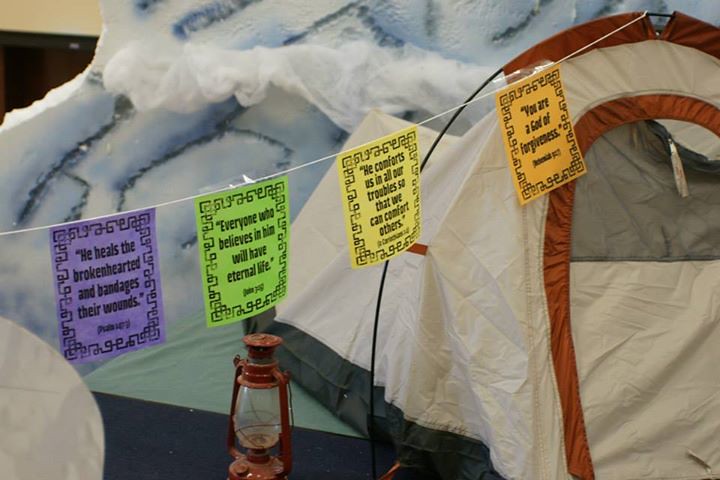This image depicts an indoor scene where a white tent with an orange zippered entrance is set up, seemingly in a living room. The tent, with its intricate foam display resembling a glacier, is positioned towards the top right of the image. Near the tent, a red lantern provides additional detail. Stretching across the center of the image is a clothesline adorned with colorful leaflets in purple, green, yellow, and orange. These leaflets display inspirational quotes with ornate borders:

- The purple leaflet quotes, "He heals the brokenhearted and bandages their wounds."
- The green leaflet states, "Everyone who believes in Him will have eternal life."
- The yellow leaflet declares, "He comforts us in all our troubles so that we can comfort others."
- The orange leaflet reads, "You are a God of forgiveness."

The background showcases a brown-bordered and white-and-blue covered tent amidst imagery of snow and ice. The setting strongly suggests an indoor arrangement, possibly evoking a spiritual or motivational ambiance.